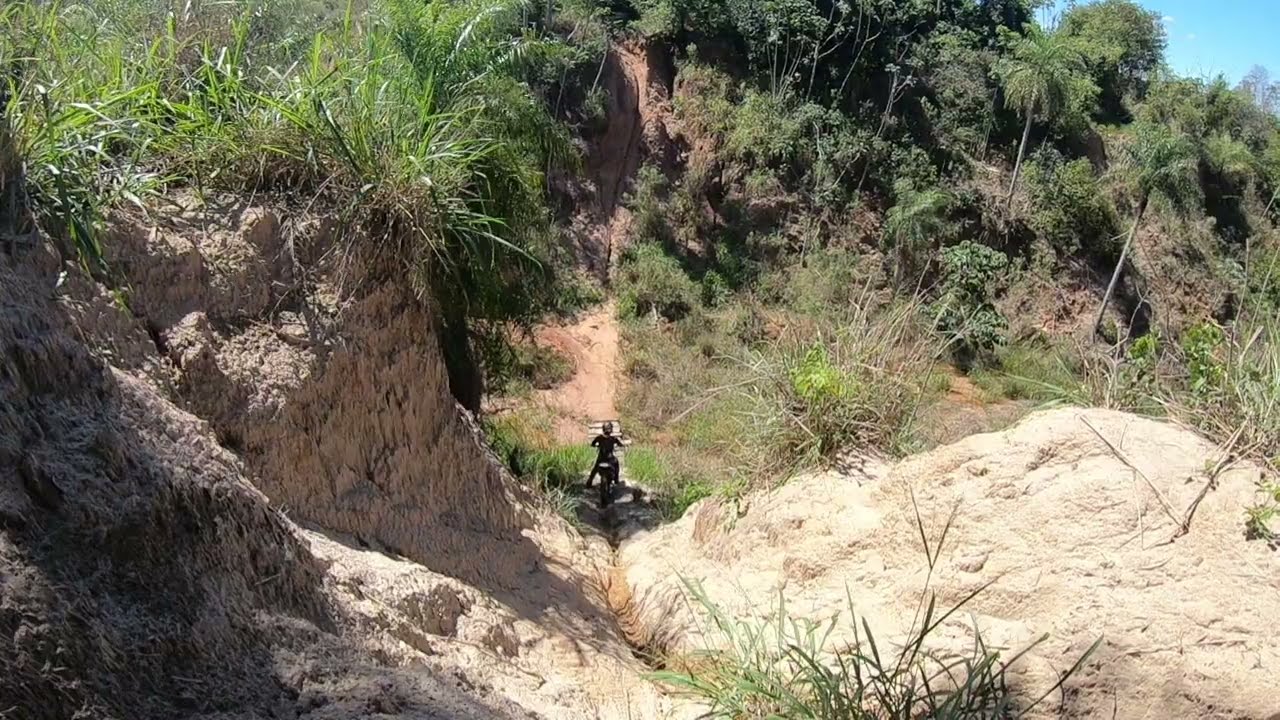The image captures a high-quality, clear view of a very narrow and precarious bike trail winding down a steep, desolate hill. The left side of the trail is lush and green, while the right side is arid, covered in sparse grass and shrubs, showcasing a contrasting terrain. In the center, at the bottom of the hill, a lone cyclist, either on a bicycle or a dirt bike, is visible, possibly having come to a stop or continuing down the trail. The trail itself extends further up another hill visible in the background. Surrounding the scene are some distant green trees under a bright blue sky, indicating a daytime setting with ample natural light. The image is presumably taken from a GoPro mounted on another bike higher up the hill, suggesting a dynamic and adventurous wilderness ride.